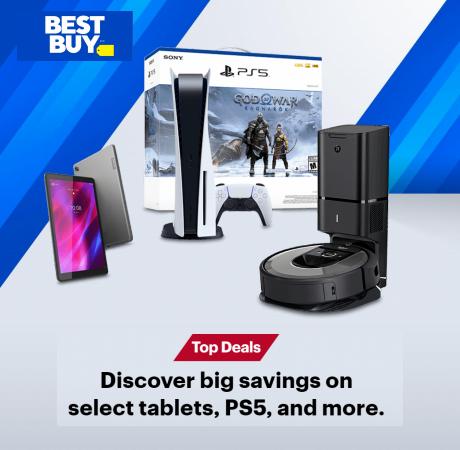This image is a detailed Best Buy advertisement featuring a selection of electronics. 

At the forefront is the PlayStation 5 (PS5), prominently displayed. The PS5 package, a white box, showcases the "God of War" video game, which features a snowy backdrop with two Viking warriors depicted in the center. In front of the box stands the PS5 console itself, an elegant tall, white tower, accompanied by a matching white handheld controller.

To the left of the PS5, two mobile phones are featured. One phone displays its screen, facing the viewer, while the other shows its sleek back design. On the right side of the image stands another electronic device, which appears to be a modern coffee maker. The coffee maker is crafted from black plastic, with a tall black tower and a flat, cylindrical base.

The backdrop of the advertisement includes blue diagonal lines running from the bottom left towards the top right, with gradient shades of blue creating a dynamic visual effect. 

In the top left corner, the iconic Best Buy logo is displayed—uppercase white letters on a blue rectangular background with a yellow price tag icon. The bottom of the image features the text: "Top Deals: Discover big savings on select tablets, PS5s, and more," emphasizing the promotional nature of the advert.